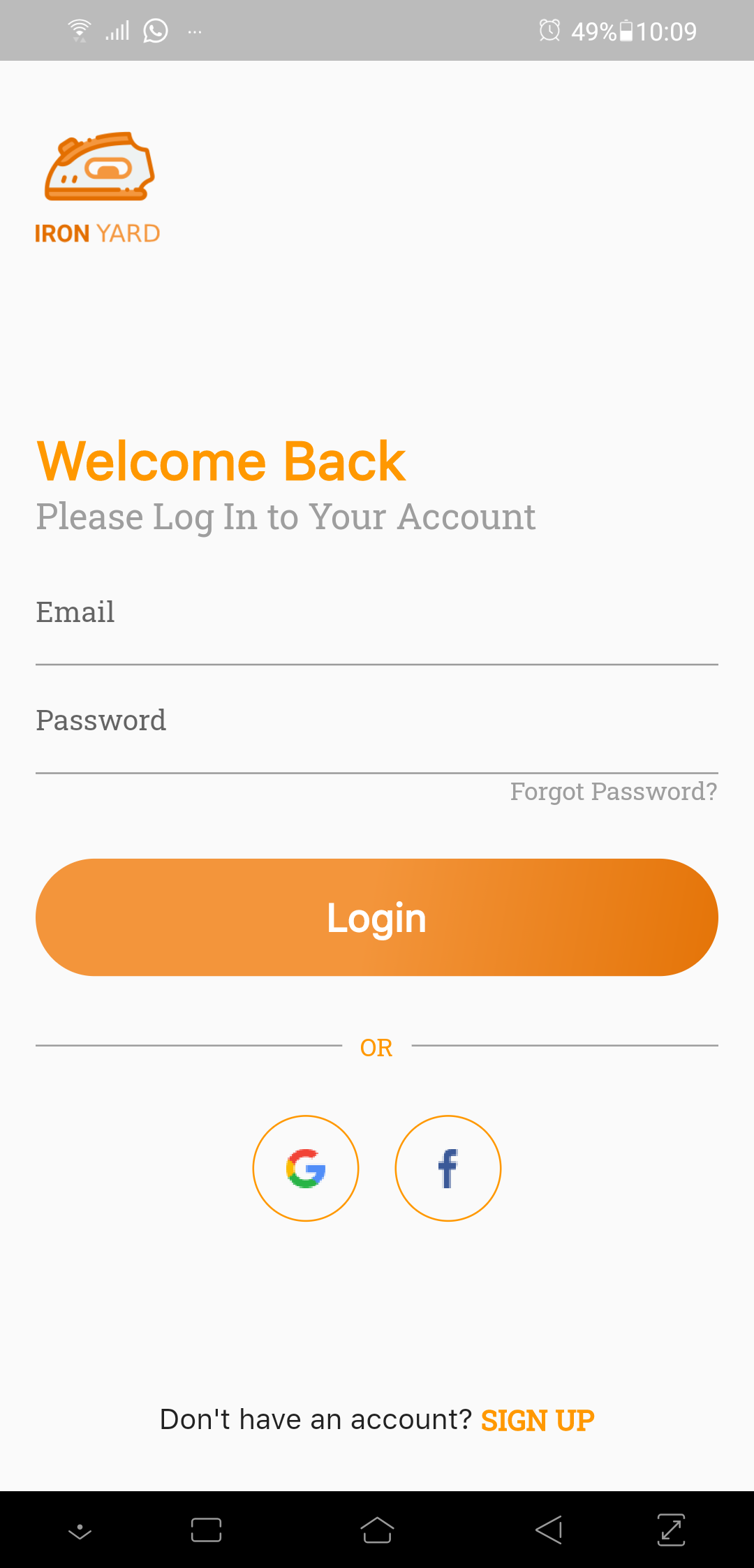This image depicts a smartphone’s screen at a specific moment, highlighting a login interface for an application called "Iron Yard." At the very top, a grey bar occupies 5% of the screen, displaying several status icons: cellular signal strength, Wi-Fi signal, a clock icon, another clock displaying the time "10:09 AM," a battery icon indicating 49% charge, and the battery percentage itself.

Below the status bar, the application’s branding is evident with an orange icon resembling an iron facing left, next to the text "Iron Yard." The interface warmly greets the user with "Welcome Back" in orange text, followed by a prompt to log into their account with the text "Please log in to your account."

The login form includes two input fields for "Email" and "Password," both of which are currently blank. To the right of the password field is a "Forgot Password?" link for password recovery.

An oval-shaped orange button with white text labeled "Log In" follows the input fields, encouraging users to proceed with the login. Beneath this button is a grey bar with the word "OR" in its center, providing alternative login options with two circular icons below it—one for Google and the other for Facebook.

Further down, amidst a section of white space, the interface queries users lacking an account with "Don't have an account?" followed by an invitation to "Sign Up" in orange text.

The bottom 5% of the screen is occupied by a black navigation bar featuring several icons: a chevron pointing down, a small box, a home icon, an arrow pointing left, and an icon that appears to increase the screen size.